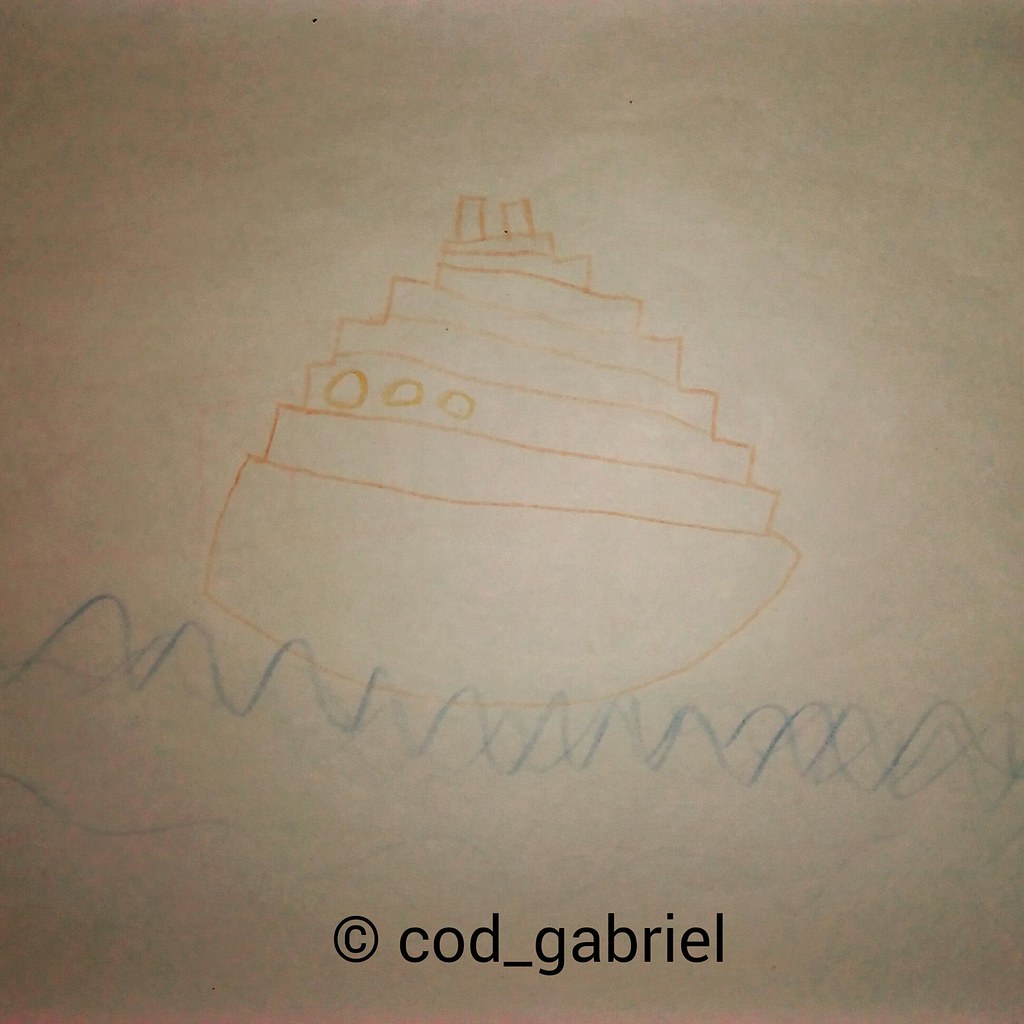This image showcases a charming, child-like drawing of a ship, likely made with colored pencils or crayons. The ship is primarily rendered in vibrant orange and displays a simplistic but endearing design. The vessel features a well-defined hull with several rectangles stacked above it, resembling either cargo containers or the multiple levels of the boat. At the top of the ship, two small chimney-like rectangles can be seen. Additionally, three tiny circles on one part of the ship suggest windows. The water beneath the boat is depicted with playful, wavy lines in blue, capturing the essence of the sea. The artwork is completed on a tan-white sheet of paper. At the bottom of the paper, a copyright note is inscribed in black, reading "COD_Gabriel."